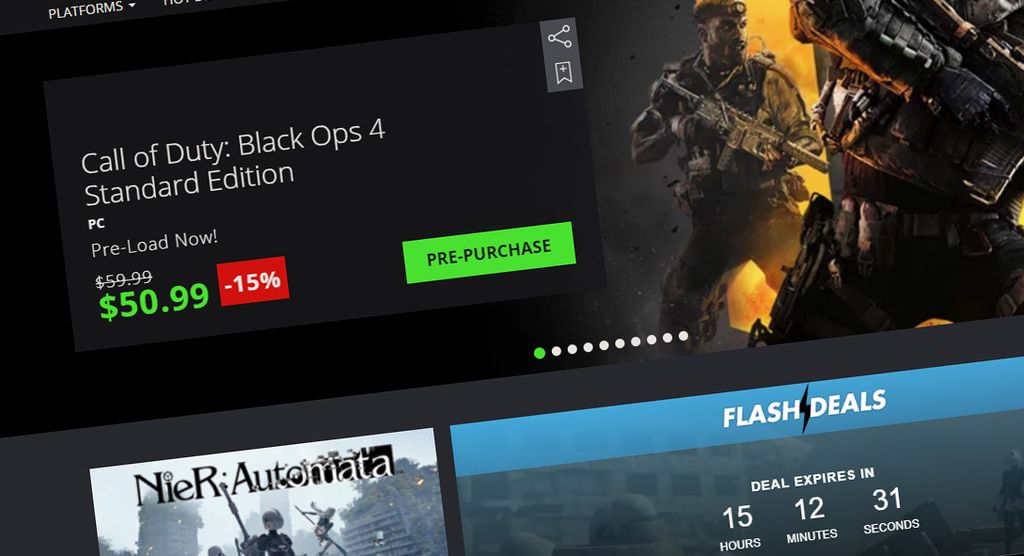This horizontal photograph captures a portion of a computer screen. The image is wider than typical landscape dimensions, approximately 35:65 in ratio. The top left corner of the screen displays a black bar with the word "PLATFORMS" in white capital letters. Below this is a gray rectangular bar featuring the text "Call of Duty: Black Ops 4 Standard Edition" alongside the label "PC, Preload Now." 

The original price of $59.99 is visibly crossed out, indicating a discount. Below it, the new price of $50.99 is shown in bold green text, accompanied by a red box highlighting a 15% discount. A green "Pre-purchase" button invites users to buy the game. An option to share this information is located on the top right-hand side of the bar.

The right side of the image partially displays a scene from the game, featuring a character in army gear, possibly wearing a beret, holding a large assault rifle. A bright yellow or fiery element illuminates the scene. Another character's back is visible, suggesting they may be reaching for their weapon, with a belt visible around their waist.

At the bottom right, a blue bar reads "FLASH DEALS" in white text, and a countdown timer shows that the deal expires in 15 hours, 12 minutes, and 31 seconds.